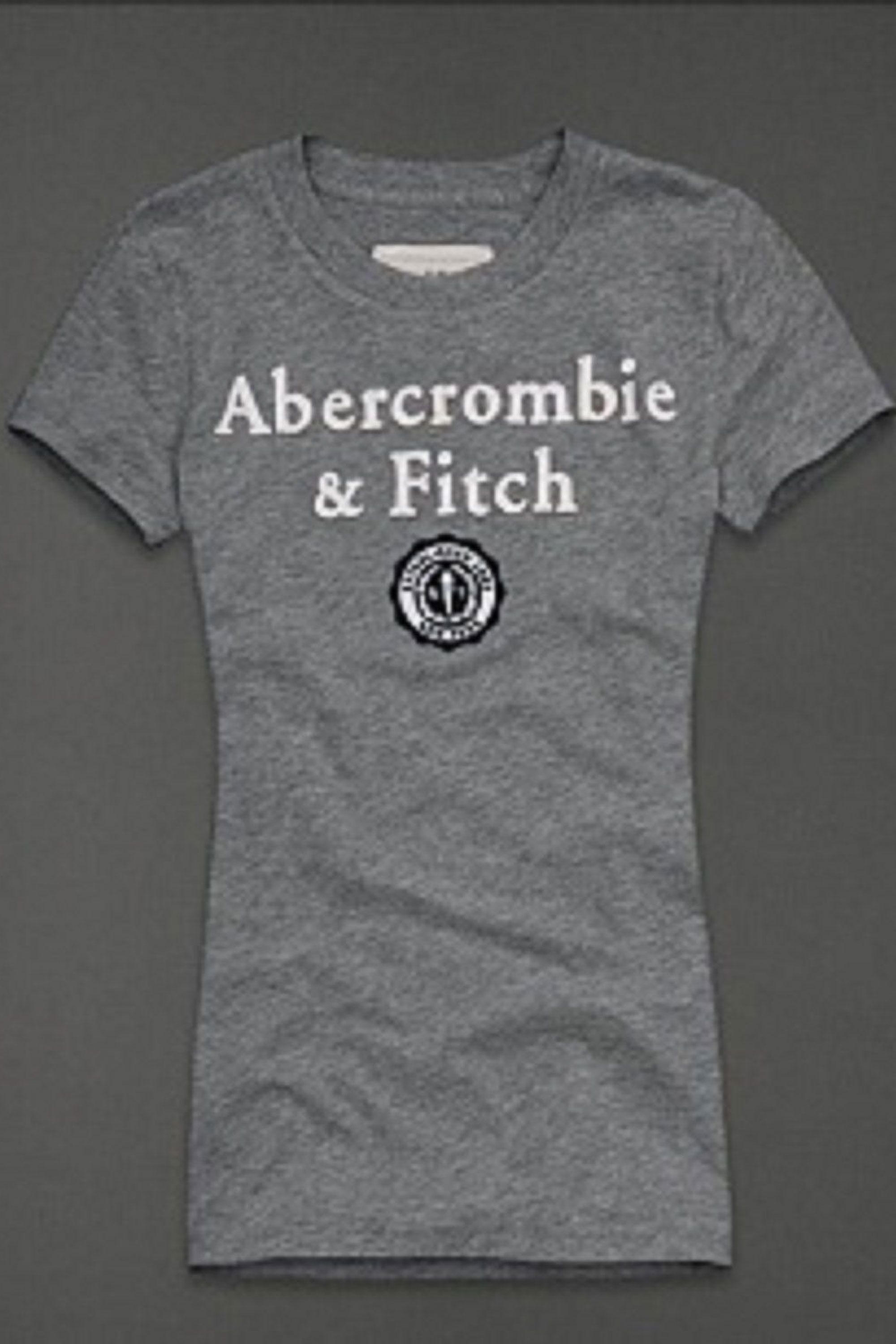This is a photograph of a narrow, light gray t-shirt with very short sleeves and a crew neck, laid out against a dark gray background. The t-shirt features large, bold white text on the front that reads "Abercrombie & Fitch," with "Abercrombie" across the top and "Fitch" beneath it. Below the text is a circular logo comprised of concentric black and white circles, although the specific details within the logo are too small to be clearly read. The fabric of the t-shirt appears slightly wrinkled. A white label with text is partially visible on the inside back of the shirt, partly obscured by the neckline.